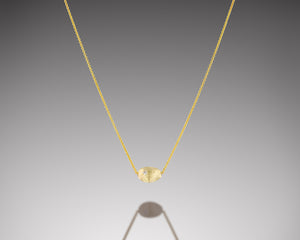This photograph captures a delicate gold necklace suspended against a subtly graded gray background that darkens at the top and gradually lightens towards the bottom. The gold chain, which is slender and appears somewhat solid rather than made of links, hangs in a long V-shape, occupying about three-quarters of the image. At the base of the V, there is a small, barrel-shaped charm that is positioned sideways, almost as if the chain threads directly through it. This charm creates a softly mirrored shadow below, mimicking its shape and slightly extending the visual harmony of the necklace in the image. The overall scene is minimalist, focusing attention solely on the elegant necklace and its intriguing shadow.